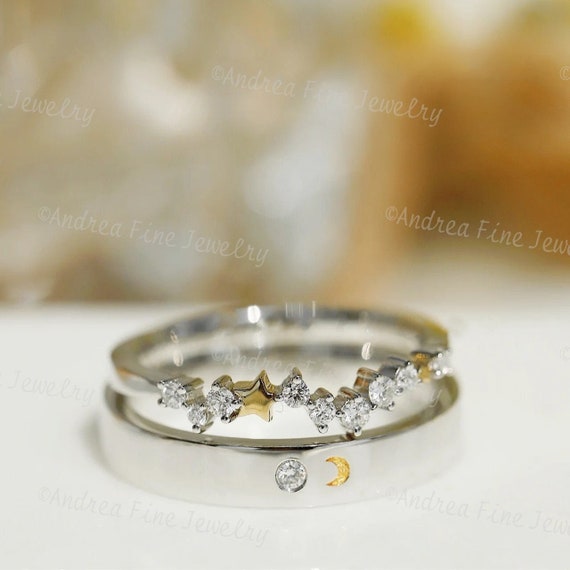This detailed image showcases an elaborate, dual-layered ring set with an astral theme. The professional promotional photo, likely from Andrea Fine Jewelry, captures a close-up macro shot with a blurred white and beige background, emphasizing the intricate details of the rings displayed atop a white cloth counter. The set appears to be composed of two distinct rings: 

The top ring, relatively thin, is crafted in silver or white gold with an irregular, starry night design. It features an array of small diamonds, probably numbering between six to nine, surrounding a singular golden star, akin to an emoji star.

The bottom ring, in contrast, is solid and thicker, also in silver. It prominently displays a single whole diamond and a yellow gemstone representing the moon. This ring complements the top ring’s celestial motif, suggesting that they are designed to be either stacked or worn together as a coordinated set. The photo focuses solely on the ring details, making it clear that this piece of fine jewelry captures the essence of the night sky with its sparkling, celestial elements.